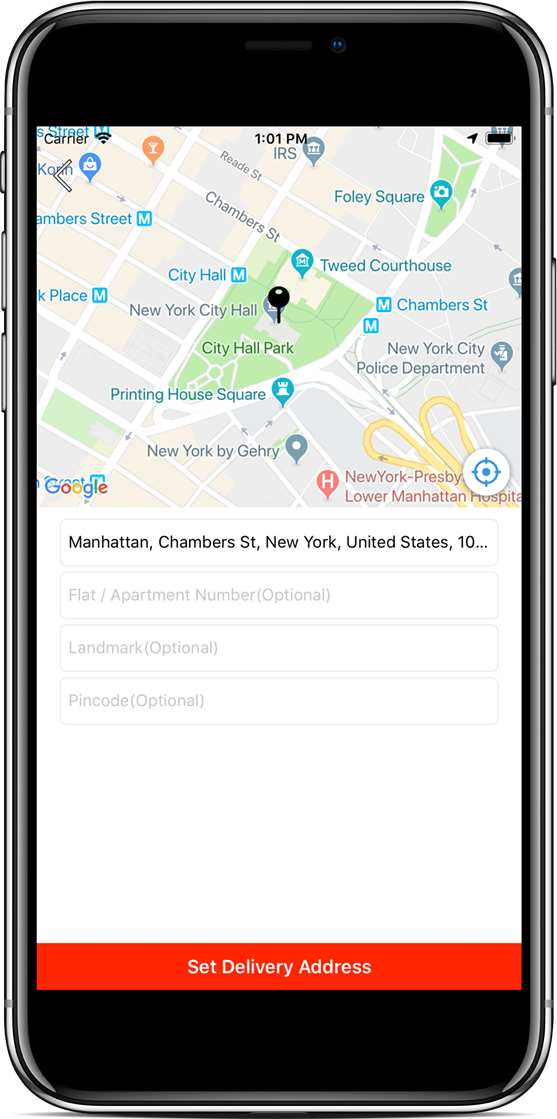The image features a modern smartphone, possibly an iPhone or an Android device. The phone has a gray bezel with a button on the upper left side and two additional buttons below it. There's also a button on the right-hand side, situated about a quarter of the way down.

On the phone's screen, a map application is open, which appears to be Apple Maps, suggested by the font used. A black bar at the top of the screen displays various status indicators: "Carrier" on the left, full Wi-Fi signal, and "1:01 PM" in the center. On the right, there is a GPS icon and a full battery indicator.

The map displayed shows a detailed section of New York City, with gray areas representing buildings and streets. City Hall Park, identified by its green color and label, is nearly in the center of the map. Various points of interest around the park are marked with gray markers, and metro lines or exits are indicated by blue "M" symbols with corresponding street names in blue text.

In the background of the map, there is a text input field where "Manhattan, Chambers Street, New York, New York, United States" is typed, along with the number "10." Additional fields for input are visible. At the bottom of the screen, a small orange bar with white text in the center reads "Set Delivery Address."